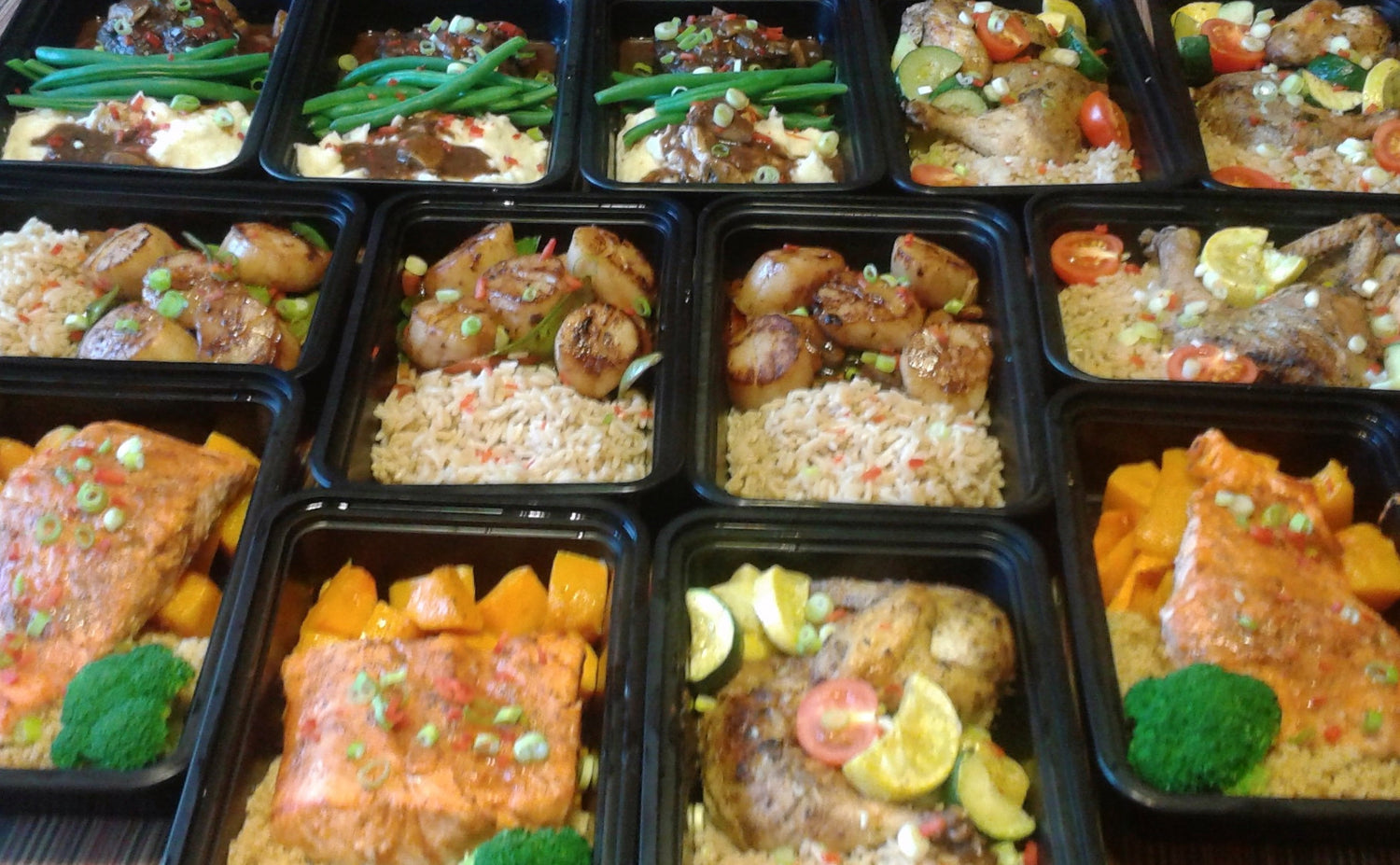The image showcases an enticing array of individually prepared meal containers, neatly organized in black trays ready for grabbing and enjoying. These meal-prepped dishes feature a variety of proteins, including seasoned chicken, fish, and scallops, paired with a selection of grains like rice and possibly couscous, giving it a Mediterranean flair. The sides are vibrant and nutritious, featuring butternut squash, zucchini, green beans, broccoli, tomatoes, and onions. One meal stands out with what appears to be mashed potatoes and gravy alongside a piece of meat. This collection of meals, resembling offerings from a meal prep or catering service, highlights an array of balanced, delicious, and visually appealing options perfect for a week of healthy eating.